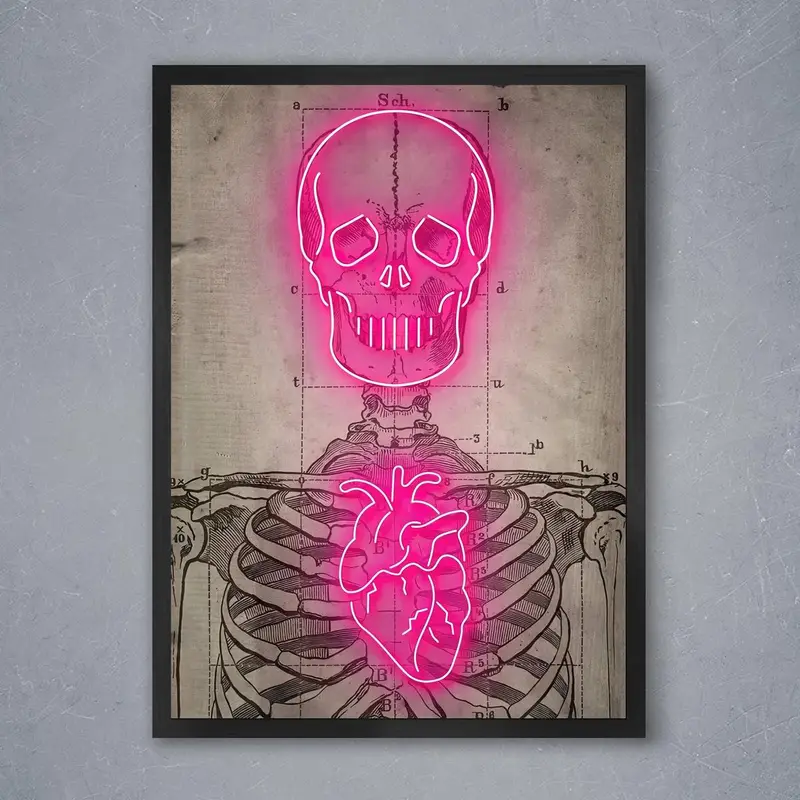This image captures a detailed framed artwork positioned against a gray wall. The black frame encases an intricate illustration of a human skeleton from a frontal perspective, rendered in monochromatic shades of black and sepia, reminiscent of an old anatomical diagram on aged paper. This diagram meticulously labels various skeletal features with lines, letters, and numbers, enhancing its scholarly appearance. Superimposed on the skeleton, vibrant neon accents add a modern twist; neon tubing outlines specific sections of the skull—highlighting the eye sockets, nasal cavity, and teeth—with glowing pink light. Additionally, an illuminated heart shape, crafted in the same neon style, is prominently depicted over the rib cage area, contrasting vividly against the sepia-toned background. This fusion of vintage anatomical drawing and contemporary neon artistry creates a captivating visual juxtaposition.